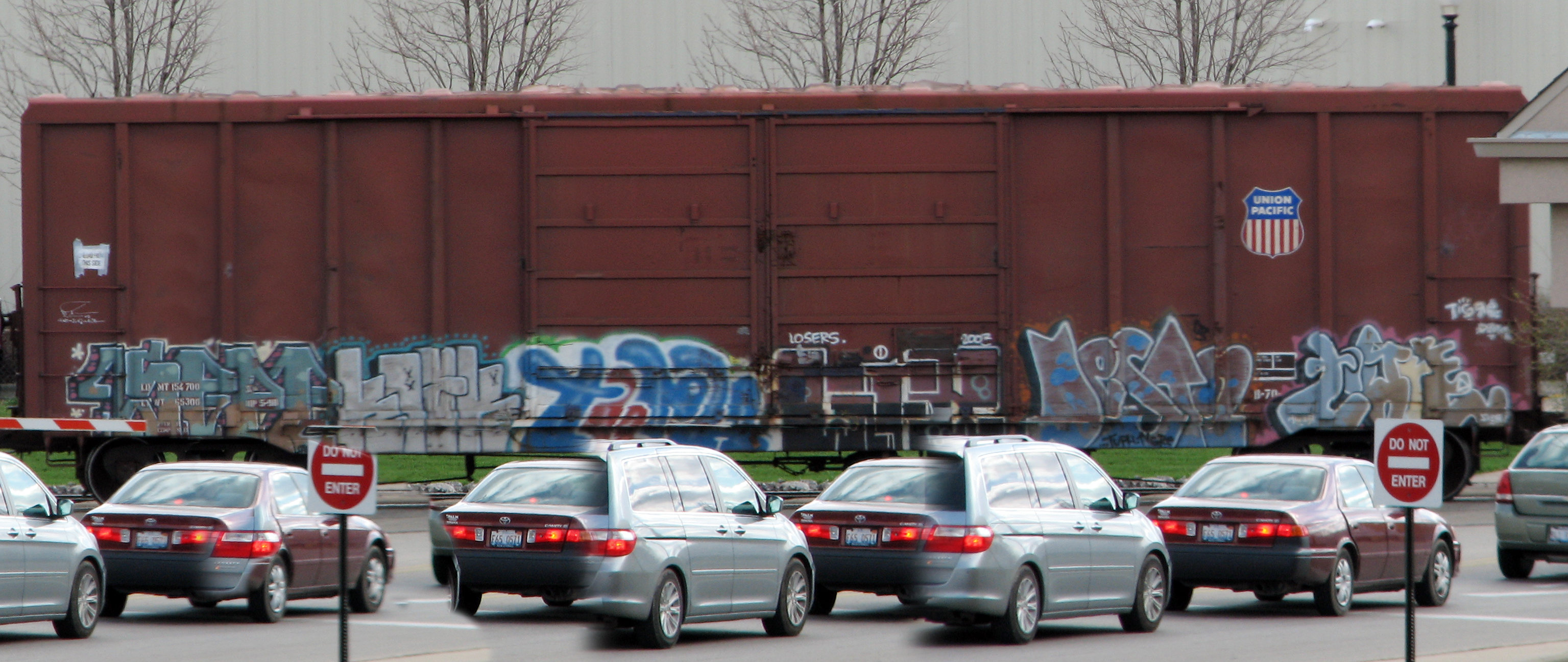This image captures a peculiar outdoor scene featuring a prominent Union Pacific train carriage set against a backdrop of four barren trees. The train, adorned with a blue, red, and white Union Pacific sign on its right side, is heavily covered in graffiti at the bottom, featuring large, unreadable block letters. In the foreground, there is an unusual depiction of traffic on a gray road. A series of vehicles is shown, but upon closer inspection, the cars appear to be superimposed and distorted, blending into each other in a glitch-like manner. This creates the illusion of multiple cars, including a gray minivan and a red sedan, merging together. Two "Do Not Enter" signs, one on each side, bracket the scene. The overall effect suggests an intentional, artistic overlay that results in repeated and morphed images of vehicles against an otherwise realistic backdrop.